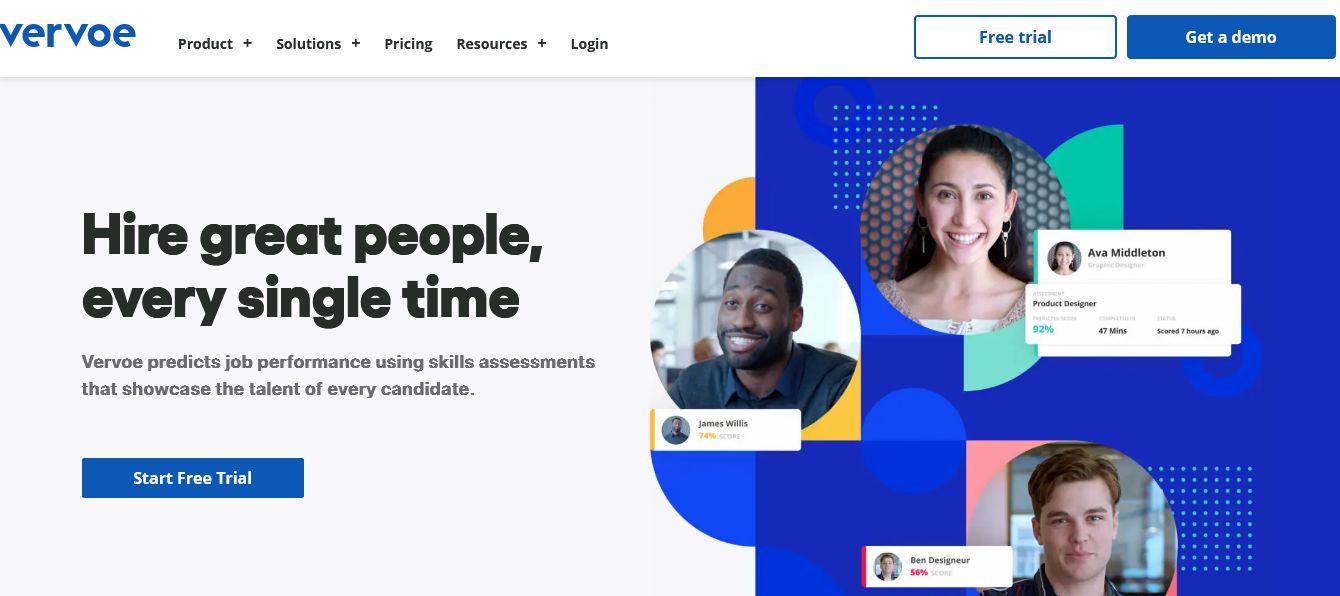This is a detailed description of a website's screenshot:

At the top left corner of the screenshot, there is a logo that says "Vervoe" in blue writing. Next to it, there are various navigation options in black writing, including drop-down menus for 'Products,' 'Solutions,' 'Pricing,' 'Resources,' and a 'Log In' button. On the top right, there is a 'Free Trial' button outlined in blue with blue writing and a 'Get a Demo' button featuring a blue background with white writing.

Below this navigation section, the left side of the screen has a grey background. On the right side, there is a complex blue background adorned with various outlined shapes such as circles, rectangles, and squares in blue, green, and shades of blue dots. Some of these shapes extend partially over the grey section on the left.

Three headshots are prominently displayed on this page. The first headshot depicts a young Asian woman with long hair. To the left is a smiling black man with short hair, a beard, and a blue shirt. Below these two is a Caucasian man with short brown hair and a subdued smile, displaying lighter skin. The text accompanying these images is too small to read.

On the left-hand side of the image, against the grey background, there is large black text that reads, "Hire great people every single time." Beneath this, it states, "Vervoe predicts job performance using skills assessments that showcase the talent of every candidate."

At the bottom of this section, there is a 'Start Free Trial' button situated on a blue background with white text.